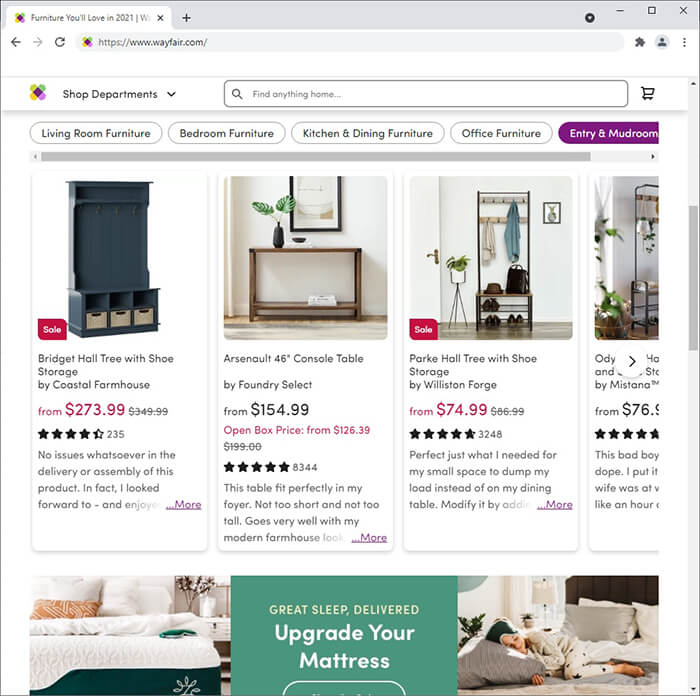The image displays the desktop homepage of Wayfair, an online furniture retailer, predominantly featuring a clean white aesthetic. The URL bar prominently shows "https://www.wayfair.com." At the top-left corner of the webpage is the Wayfair logo. Beside it, there's a "Shop Departments" button with a small arrow indicating a dropdown menu for expanded options. To the right of this is a search bar and a shopping cart icon.

Below the primary navigation section is a horizontal menu with various category options including "Living Room Furniture," "Bedroom Furniture," "Kitchen and Dining Furniture," "Office Furniture," and "Entry and Mudroom." The "Entry and Mudroom" category is highlighted in purple, indicating it has been selected.

Displayed prominently in this category is a selection of items starting with a Bridget Hall Tree with shoe storage, showcasing a blue storage solution for shoes, complete with a price, star rating, and a snippet of a customer review. The subsequent items listed include a console table, another shoe storage unit, and a partially visible fourth item that also appears to be related to shoe storage.

Towards the bottom of the webpage, there's a partially visible banner related to mattresses. The banner features an image of a bed with someone sleeping on it, complemented by text indicating a promotional message: "Great Sleep Delivered. Upgrade Your Mattress."